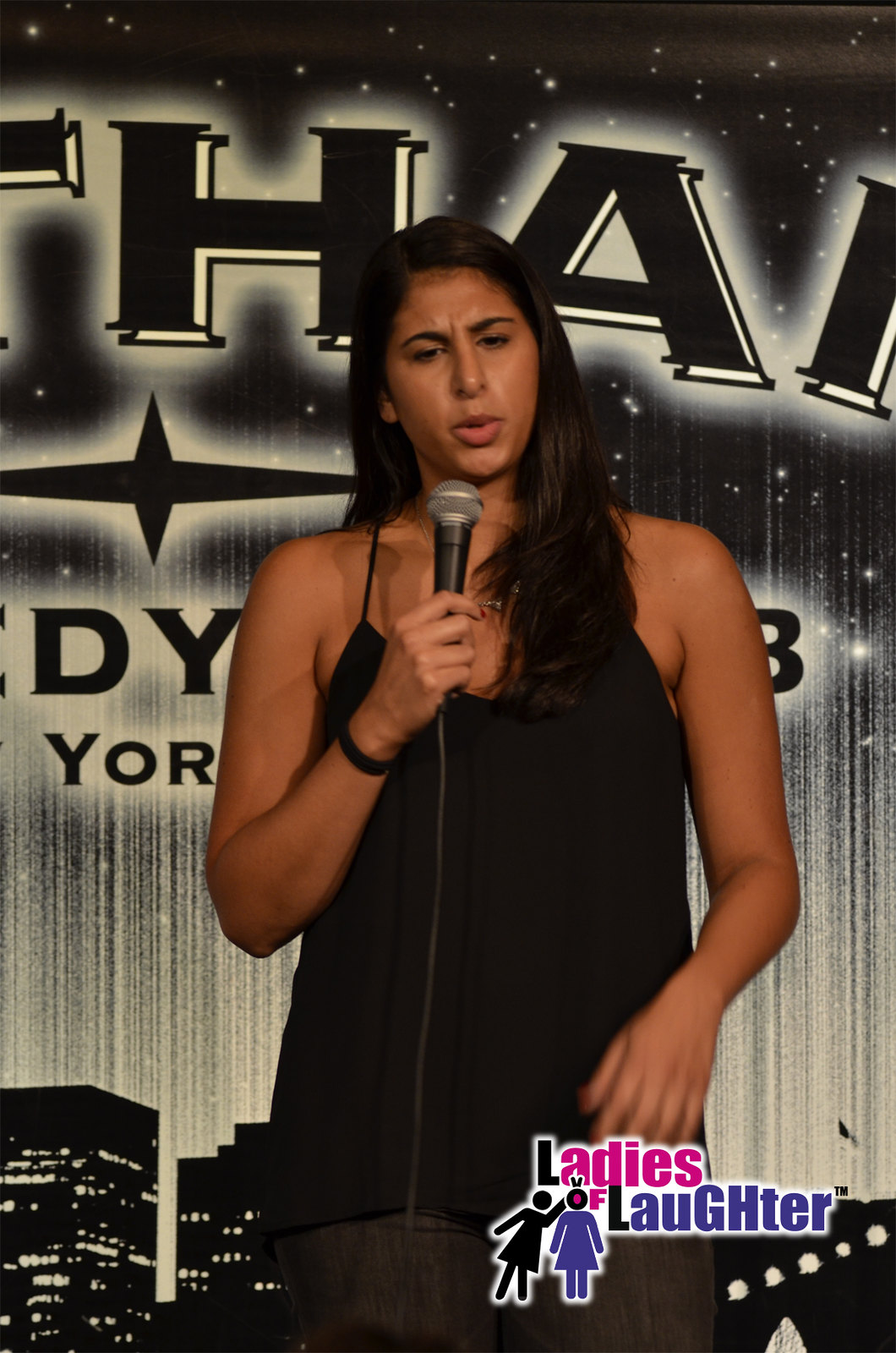In the image, a young woman with long brown hair is on stage, holding a microphone and addressing the audience. She appears to be in her late 20s or early 30s, dressed in a black spaghetti-strap top and black pants. A stage backdrop features a city skyline with black office buildings lit up against a cloudy white sky. The top of the backdrop shows large black letters outlined in white, though the full wording isn't visible. Below these letters, there's a prominent four-pointed star and partial letters that suggest the venue might be in New York. An icon at the bottom of the backdrop promotes 'Ladies of Laughter' with the text 'Ladies' in pink and 'Laughter' in purple. This icon includes silhouettes of two women, one in black and one in purple, against a white background, with one woman leaning into the other. The young woman on stage seems to be engaged in either singing or stand-up comedy, contributing to a lively and engaging atmosphere.